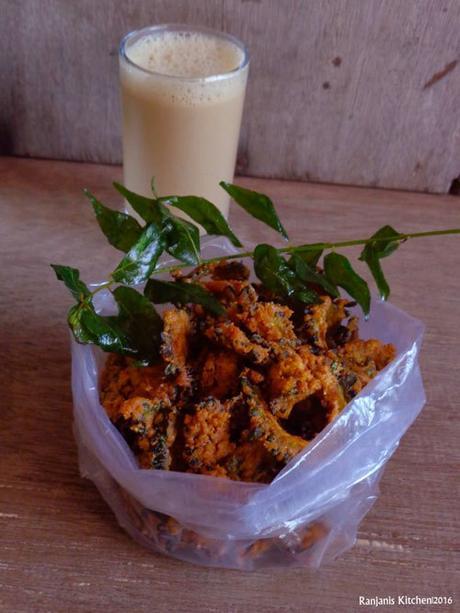In "Rajani's Kitchen, 2016," the foreground showcases a clear plastic bag brimming with medium-brown, curled, fried foods resembling rings or possibly shrimp. Perched atop the fried items is a thin branch with greasy green leaves, adding a decorative touch to the presentation. The bag rests on a brown wooden surface that forms a slight angle with the gray wooden wall in the background. Behind the bag, a glass of almost full, foamy white liquid—likely milk or a light chocolate milk—completes the setup. This rustic and thoughtfully arranged scene highlights an inviting blend of crunchy textures and refreshing drink.